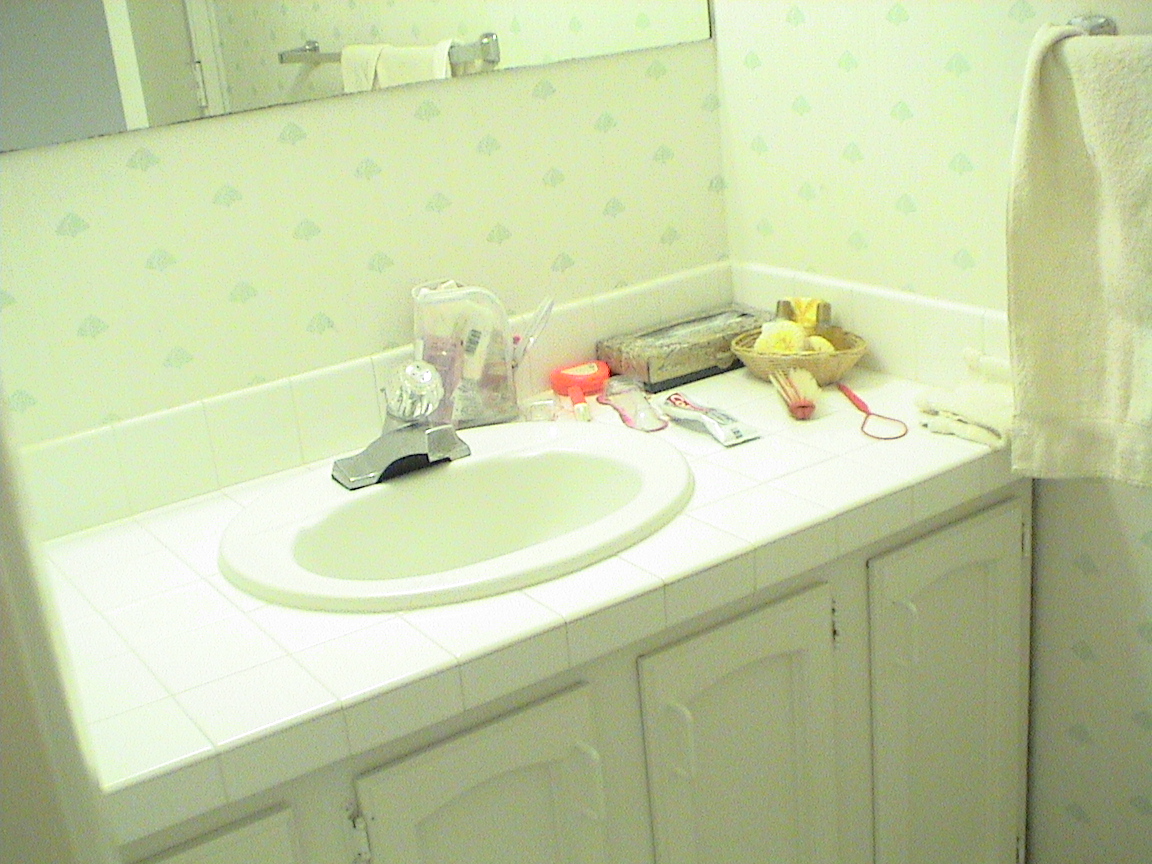A vintage 1980s bathroom is depicted in this image, characterized by several distinct features. The sink features a unique faucet with a clear globe handle that you pull up and twist to control the water flow. Both hot and cold water come out from a single spout. The sink itself has a substantial lip outlining it, and it's painted in a dated greenish hue. The countertop, likely tiled, appears to be a mix of green and light beige, or possibly off-white. In one corner of the countertop, there is a tissue box and a basket holding various toiletries. Scattered across the countertop are a hairbrush, toothpaste, and a bag of toiletries positioned behind the faucet. A towel hangs loosely on the rack, not folded. Beneath the sink, there is cabinetry with old-fashioned pulls and doors, consistent with the age of the bathroom. The wallpaper is very dated, in a cream or green color with some sort of green design. The basic mirror above the sink is discolored around the edges, adding to the bathroom's aged appearance. In the reflection of the mirror, an old and discolored door is also visible.